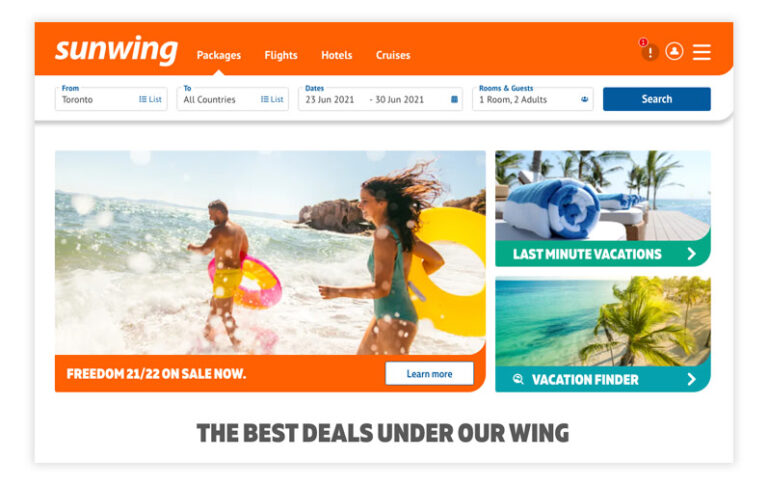At the top of the image, there's an orange banner featuring the text "Sunwink Packages" in white. Beneath it, a section highlights various travel options including flights, hotels, and cruises. 

Below this banner are several rectangular sections with gray borders and white interiors. The first rectangle details a travel itinerary: "From" in blue followed by "Toronto" in black; "List" in blue; "To" in blue followed by "All countries" in black; "List" in blue; "Dates" in blue stating "23 June 2021 to 30 June 2021" in black; "Rooms and Guests" in blue with "1 room, 2 adults" in black. A navy blue "Search" button, written in white, concludes the section. 

The central part of the image contains several pictures. The first image depicts two people running into the ocean, each holding inflatable pool donuts, one yellow and one yellow and pink. An orange border frames this picture with "Freedom 21, 22 on sale now." written in white. Beneath this text is a blue "Learn more" prompt.

To the right, another image showcases towels near palm trees by the water. This image is highlighted by a green rectangular background with "Last-minute vacations" written in white.

Below these images, an aerial view of a beach and trees is provided. This image is framed by a teal border with "Vacation Finder" in white. Below it, in dark gray, the caption reads, "The best deals under our wing."

At the very bottom of the image, all these visual elements are consolidated, concluding the travel-themed display by Sunwink Packages.